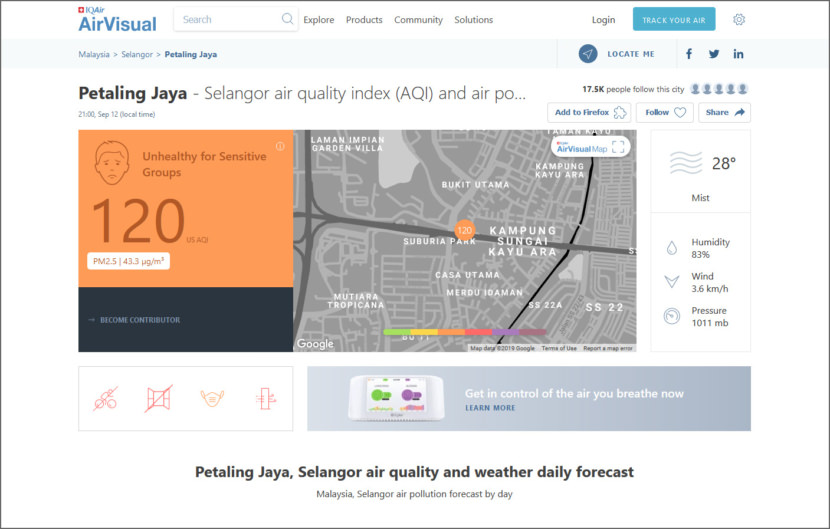A screenshot of the AirVisual web page displays a multitude of features and data related to air quality and weather. At the top of the page, there is a search bar accompanied by navigation options including "Explore Products," "Community Solutions," "Log In," "Track Your Air," and "Settings." The location hierarchy is shown as "Malaysia > Selangor > Petaling Jaya," with a "Locate Me" function provided. Social media icons for Facebook and Twitter are present, alongside buttons to "Add to Firefox," "Follow" (denoted with a heart icon), and "Share" (represented by an arrow icon).

The air quality status for Petaling Jaya, Selangor is prominently displayed with a rating of 120, categorized as "Unhealthy for Sensitive Groups." This is visually reinforced by an icon of a person with a sad face on an orange square background. To the right, a grey and white layered street map of the city is featured.

Additional weather information includes an air symbol indicating misty conditions, a temperature of 28 degrees Celsius, 83% humidity, wind speed of 3.6 kilometers per hour, and air pressure at 1011 MB. 

Below this, the page offers a daily forecast for Petaling Jaya, highlighting both air quality and weather forecasts. The page encourages users to take control of their air quality with a prompt to "Learn More."